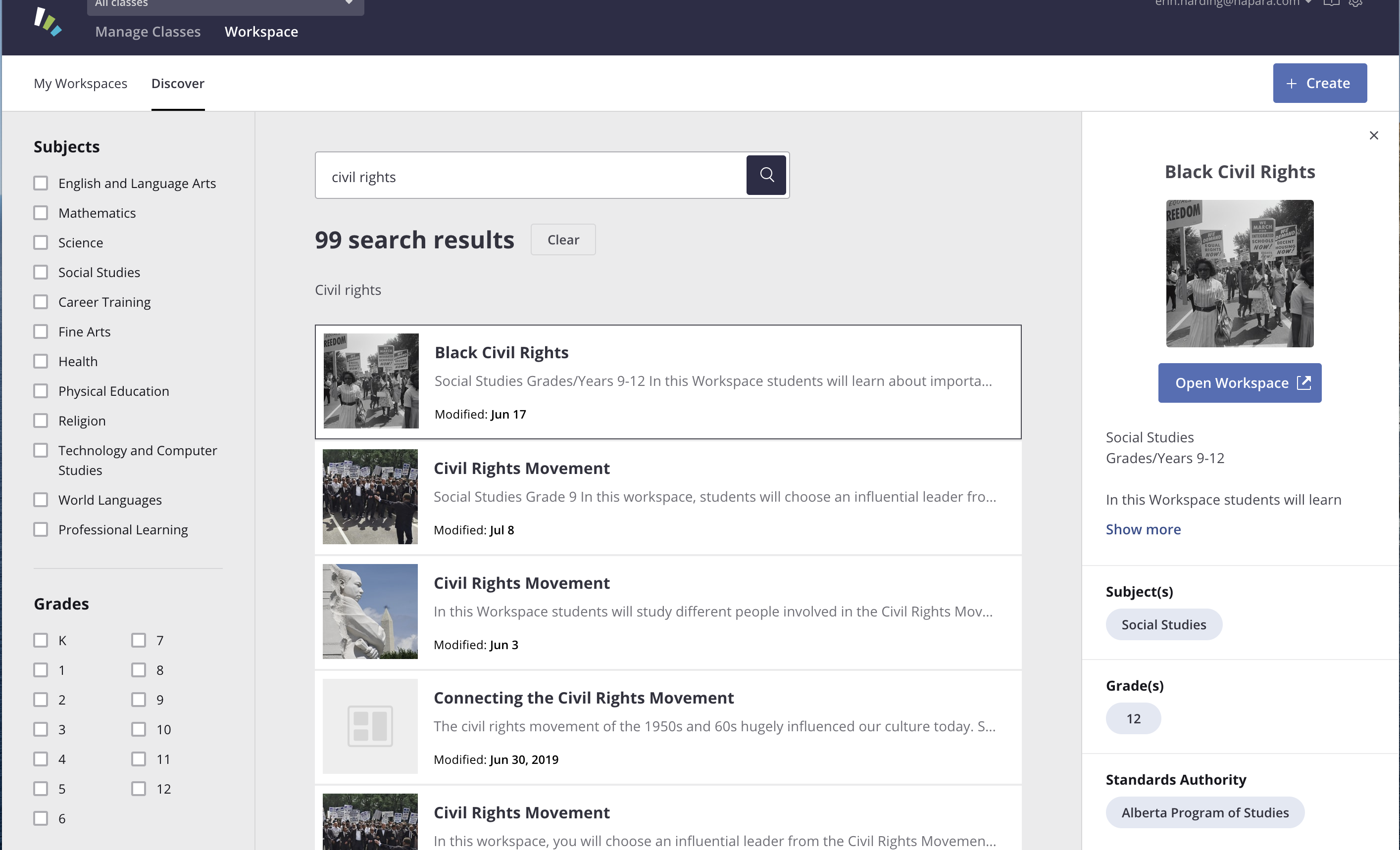This screenshot depicts a user interface of an educational or workplace platform designed for managing and discovering various resources. On the left side of the screen, a sidebar is titled "My Work Spaces," and adjacent to it is a "Discovery" tab. Dominating the top portion, there is a blue header displaying "Manage Classes Workspace." Below the "My Workspace" and "Discovery" tabs, a "Create" button is visible, signifying an option to create new workspaces or content.

Underneath the "Create" button, there is a list labeled "Subjects," featuring diverse categories such as English and Language Arts, Mathematics, Science, Social Studies, Career Training, Fine Arts, Health, Physical Education, Religion, Technology and Computer Studies, World Languages, and Professional Learning. Adjacent to this list, a section titled "Grades" encompasses the entire K-12 spectrum.

In the central part of the screen, a search functionality is engaged, with the term "Civil Rights" entered. The search results yield 99 entries, starting with topics such as "Black Civil Rights," "Civil Rights Movement," another entry named "Civil Rights Movement," followed by "Connecting the Civil Rights Movement," and yet another "Civil Rights Movement." Four of these entries include an accompanying image.

On the far right, a preview panel showcases the details of the first search result, "Black Civil Rights," specifying it as a Social Studies resource suitable for grades 9 to 12. There is an option to open the corresponding workspace for further exploration.